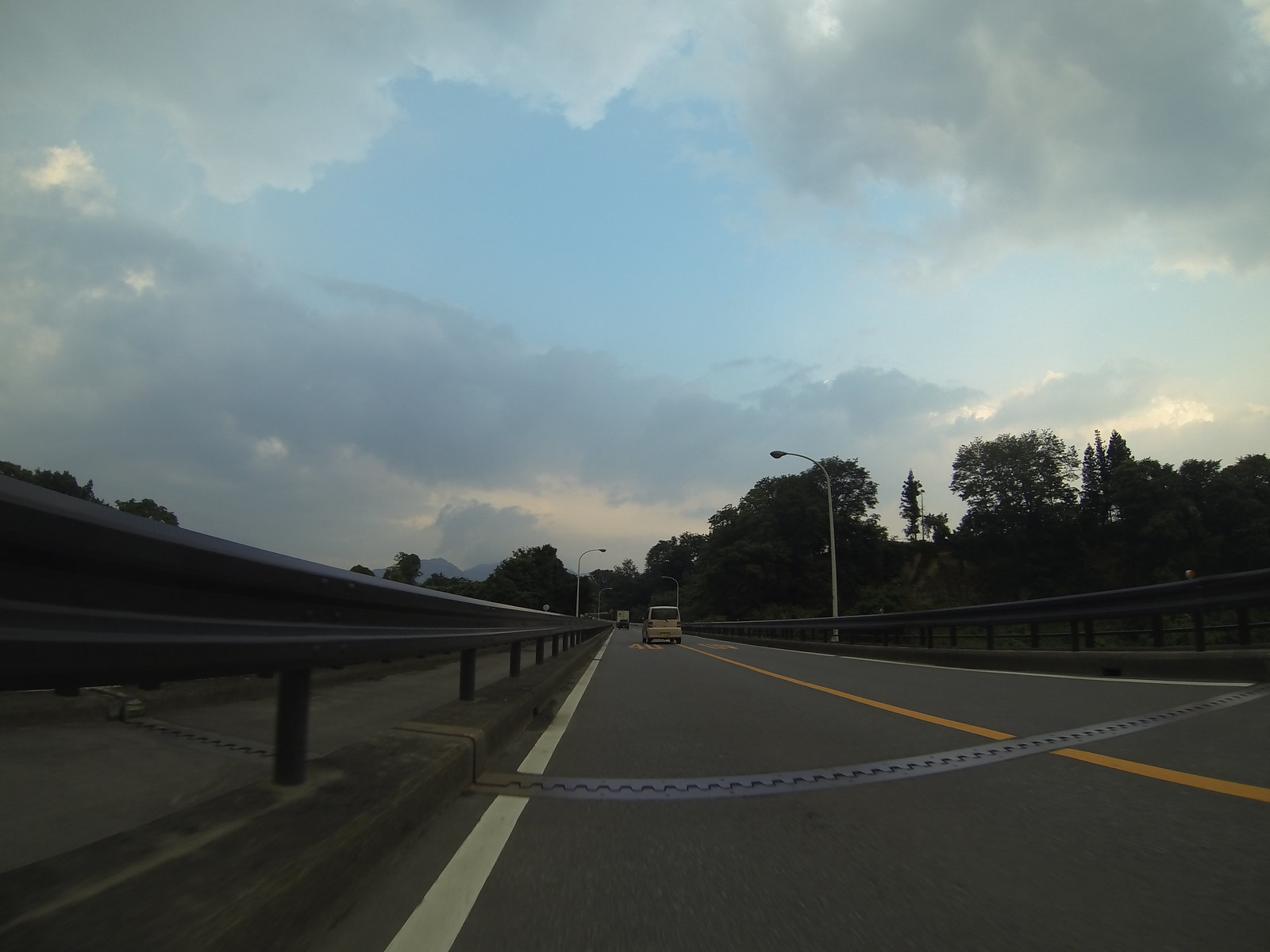The image captures a scenic roadway under a dramatic sky. The expansive sky showcases a palette of colors, with a soft blue that becomes lighter towards the right, suggesting the presence of the sun. This illumination hints at the early stages of sunrise or the dwindling light of sunset. Scattered throughout the sky are numerous clouds, ranging from darker, grayish tones to lighter patches illuminated by the sun.

Just below the sky, a road stretches into the distance. The perspective is from a low angle at the bottom of the road, allowing a close-up view of its features. Yellow lines mark the center of the pavement, guiding the way forward. On the sides of the road, barriers provide a sense of safety, while a square-shaped car drives away, enhancing the depth of the scene.

Adjacent to the road on the left is a sidewalk, providing a contrasting element of structure. The right side of the road is bordered by an array of trees, adding a touch of nature to the setting. Light posts are staggered along the roadside, hinting at the onset of evening or morning, ready to illuminate the scene as needed.